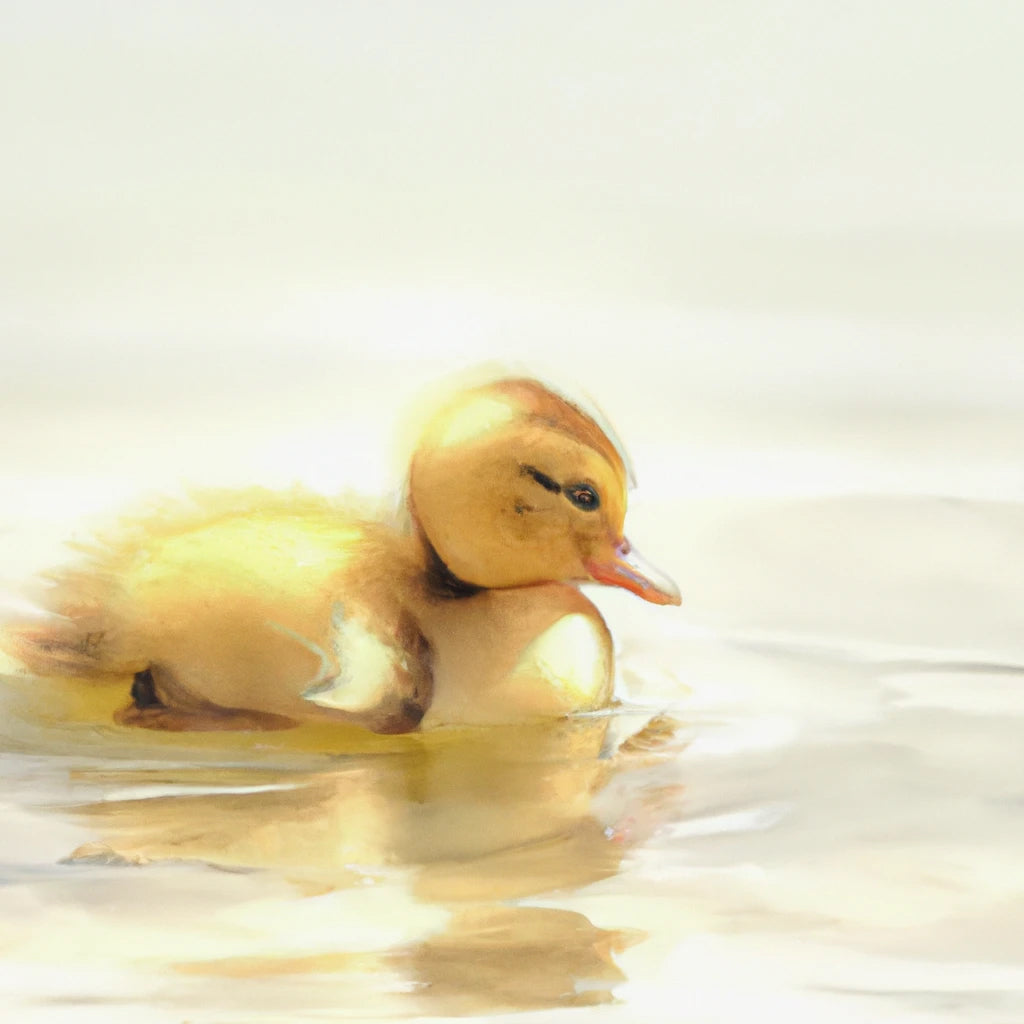The image depicts an adorable baby duckling, rendered in a watercolor painting style, floating serenely on a pond. This small, fluffy duckling is a light yellow color, with a pale orange beak and a distinctive black eye. Its soft, fuzzy down covers its back and head, giving it an endearing youthful appearance. The duckling's head is slightly tilted downward, creating a content and peaceful expression, almost as if it's smiling. The water beneath it is a blend of beige and gray hues, with gentle ripples emanating from the duckling, suggesting a subtle movement. There's also a faint reflection of the duckling in the water, although it isn't very clear. The background of the painting is a muted, greenish-white, possibly representing a bright sky. The entire scene exudes a calm and neutral ambiance, making it an ideal piece for a nursery.